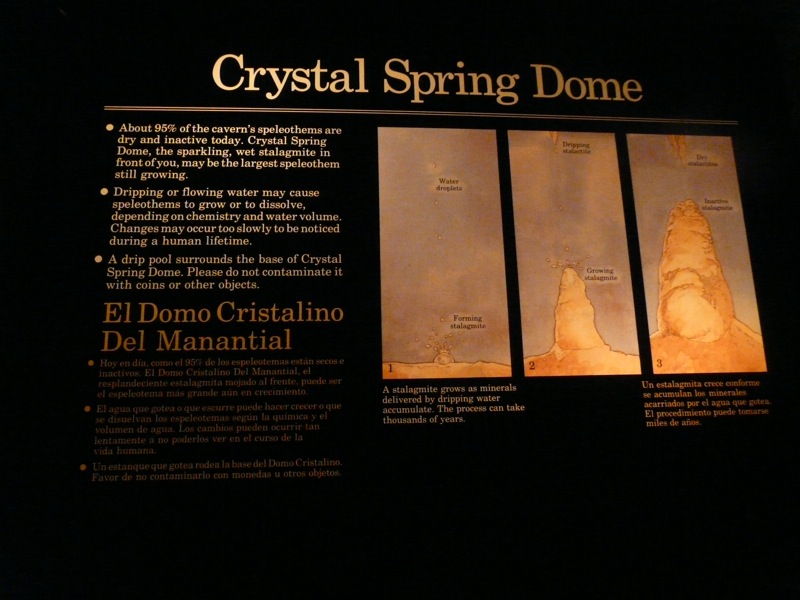The image shows a detailed informational plaque predominantly surrounded by a black background with elegant gold writing. At the top, in bold letters, it reads "Crystal Spring Dome." Below this title is a sequence of three gold illustrations resembling termite mounds, increasing in size from left to right. These images are indicative of the growth stages of speleothems, presumably stalagmites or stalactites, rising from the ground towards the sky.

To the left of these images, the plaque provides several informational points in gold text. It explains that about 90-95% of the cavern’s speleothems are currently dry and inactive. Some text notes that the Crystal Spring Dome is a sparkling, wet stalactite which may be one of the largest speleothems still actively growing. Another point emphasizes the role of dripping or flowing water in the formation or dissolution of speleothems, stating that changes tend to be so gradual that they go unnoticed within a human lifetime. Additionally, there’s a cautionary note advising visitors not to contaminate the drip pool at the base of the Crystal Spring Dome with coins, objects, or other pollutants.

At the bottom of the plaque, there is some additional smaller gold writing, with one notable phrase being "El Domo Cristalino del Manitano," repeated in Spanish along with other text too small to read. 

Overall, this plaque serves as an educational guide, likely located within a cave or cavern, detailing both the specifics of the Crystal Spring Dome and general speleothem formation processes.